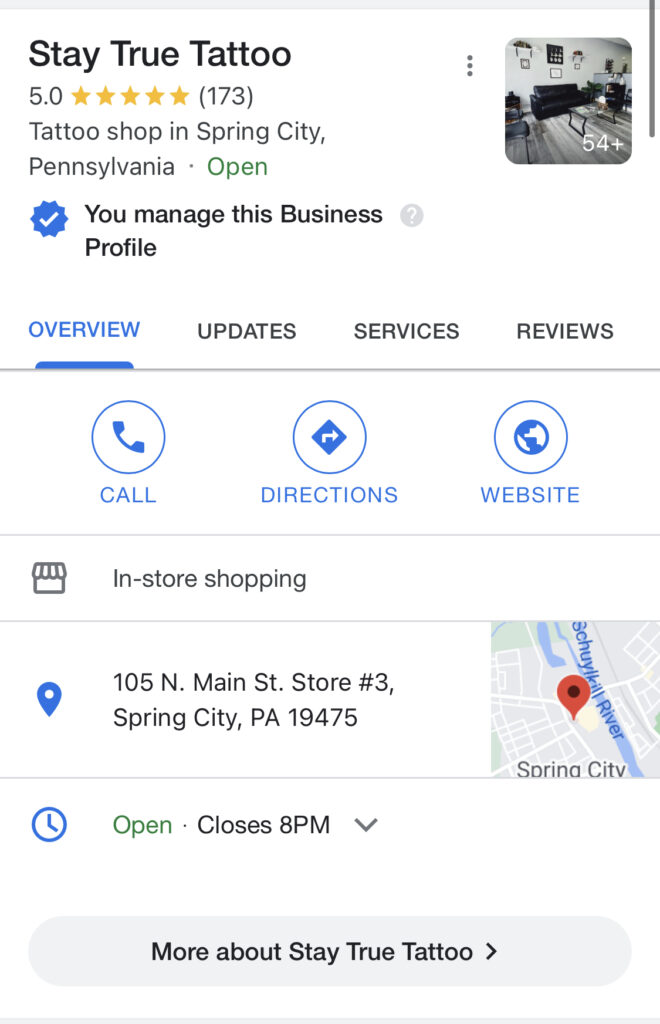Here is a cleaned-up and detailed caption for the image:

---

This screenshot showcases the review page for Stay True Tattoo, a tattoo shop located in Spring City, Pennsylvania, which boasts an impressive 5-star rating based on 173 reviews. The page is managed by the business owner, as indicated by the blue checkmark and the tag "You manage this business profile." The profile features a cover photo of the tattoo parlor and includes a collection of 54 images.

Prominently displayed at the top are four navigational tabs: Overview, Update, Services, and Reviews. Below these tabs are three action buttons: Call, Directions, and Website. The shop's address is listed as 105 North Main Street, Store Number 3, Spring City, Pennsylvania, 19475. The business hours are provided, noting that Stay True Tattoo closes at 8 PM. 

A map is embedded on the page, pinpointing the exact location with a red location marker. A bolded section at the bottom urges visitors to learn more about Stay True Tattoo. The user interface is primarily white, with a visible scrollbar on the top right.